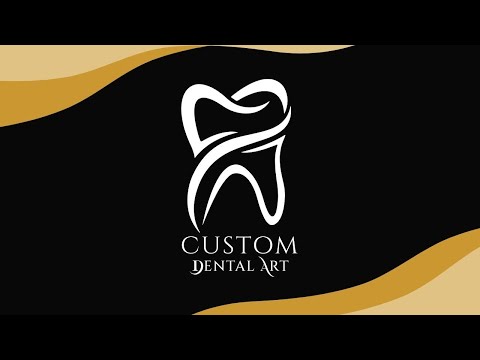This rectangular corporate logo for Custom Dental Art features a modern, stylized white tooth emblem composed of four curved, swirling segments, set against a solid black background. The intricate tooth design gives it a sleek and appealing look. The logo is accompanied by the text "CUSTOM DENTAL ART" in unique, uppercase white block font, positioned below the tooth graphic. Adding to the visual interest, two-tone yellow ribbons with wavy, sinusoidal borders frame the image, extending from the upper left to the lower right and vice versa. These ribbons come in light yellow and a darker mustard yellow shades, enhancing the overall aesthetic of the image. The black background extends slightly beyond the image's borders, creating a clipped effect on the top and bottom, giving the logo a polished and professional appearance.